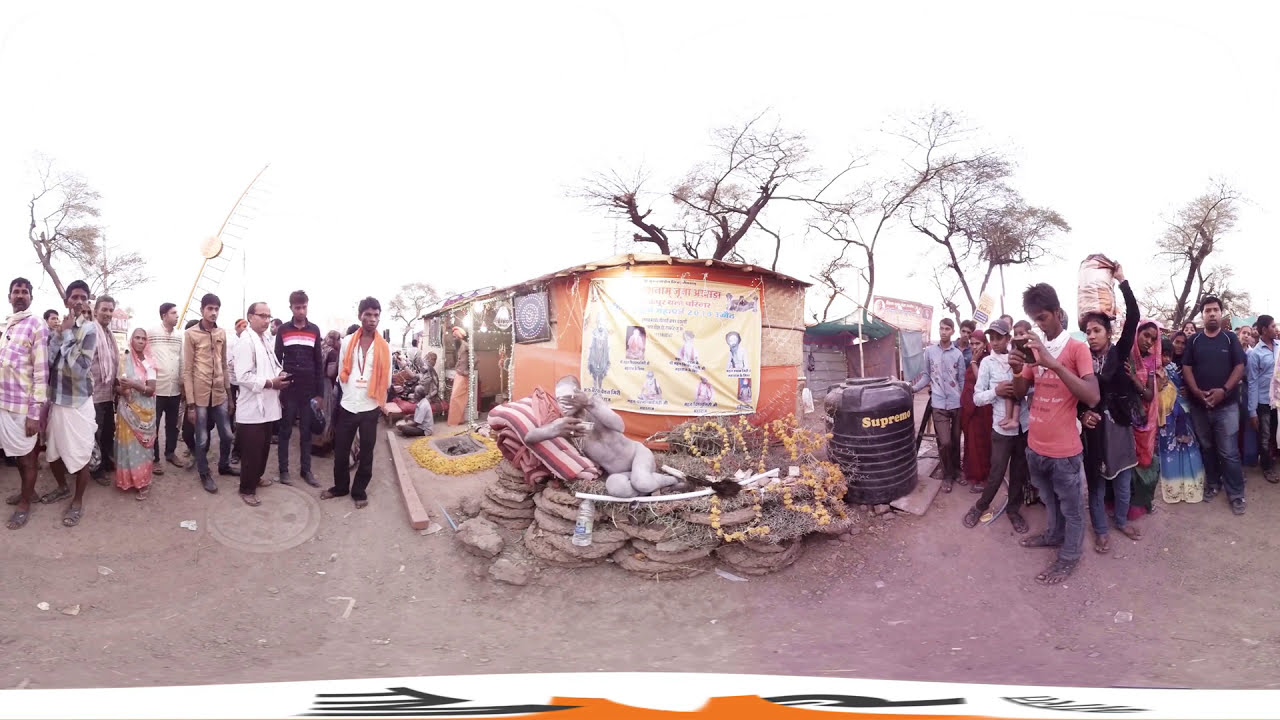The photograph captures an outdoor scene in another country, characterized by an overcast, white sky and a dirt ground with sparse, nearly leafless trees, giving it a desolate, desert-like appearance. A small crowd of people, including a doctor, surrounds a main focal point: a person who appears to be nude and is covered in a white clay substance, positioned on a pink and red comforter atop what looks like dried mud paddies. This person is holding a water bottle, adding to the realism of the scene. The onlookers have brown skin, are dressed in colorful garments such as dresses, saris, plaid shirts, white shorts, and long tunics, and many are either barefoot or in open-toed sandals. Some people are looking at their phones while others are gazing intently at the central figure. There's an orange shanty-style building with a white banner, adorned with blue and orange markings and pictures, though the text is unreadable due to the bright light above it. The atmosphere suggests a mix of anticipation and curiosity, with elements hinting at a marketplace setting. Scattered around are various items, including what appears to be a trailer filled with miscellaneous things, further contributing to the scene's cluttered appearance. This detailed combination of human activity and environmental details underscores a complex and intriguing moment captured in the photo.